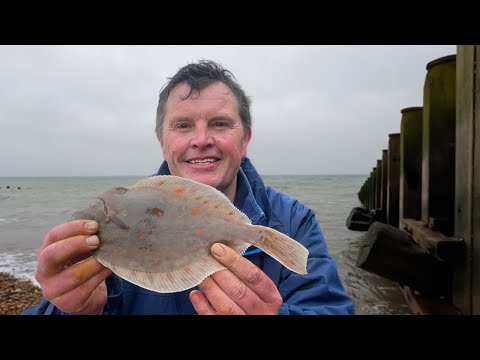In this image, a man stands proudly at the center, holding a flat, gray flounder with distinctive orange polka dots. He wears a blue jacket and has a content, relaxed expression on his slightly weathered face, suggesting he is in his mid-fifties. His gruff hands with dirty fingernails emphasize his outdoorsy nature. The background reveals a grayish white sky over a grayish green ocean, with rocky beach waves crashing behind him. To the right, a row of wide, rectangular wooden logs forms a pier that stretches out into the water. The man's receding hairline and thinning hair on top and sides are visible, adding a touch of character to his joyful disposition.